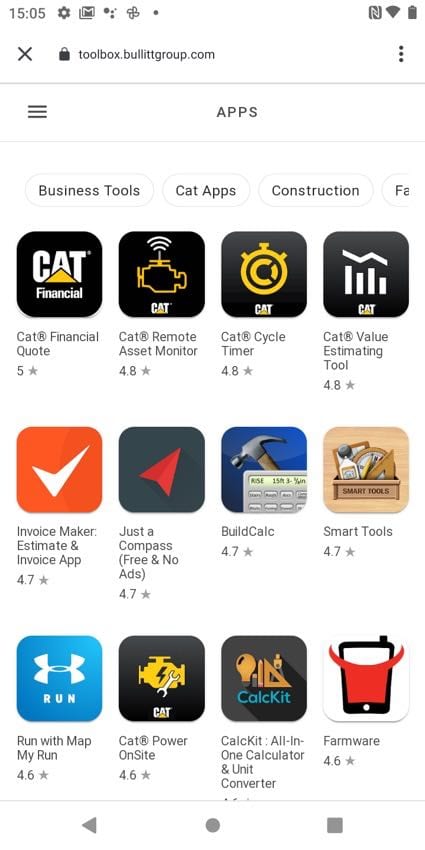**Detailed Caption:**

The top of the interface lists a sequence of icons and symbols including "1505," a gear, a "Gumo" symbol, a fan, an NFC icon, a Wi-Fi signal, a battery indicator, an "X" symbol, a lock, a toolbox, and a partially obscured website URL "toolbox.bulletgroup.com...". A hamburger menu is present, alongside an assortment of app categories and tools. Under the "Business Tools" section, the categories are "Cat Apps," "Construction," and a black square labeled "Cat." Additionally, there are payment and financial tools such as "Cat Financial Quote" rated 5 stars. 

Other tools and apps listed involve functionalities like remote management, indicated by icons such as an engine, Wi-Fi signal, and thermometer. Specific apps include "Cat Cycle Timer" rated 4.8 stars, "Lines and Bar" rated 4.8 stars, and "Cat Value Estimate Total" also at 4.8 stars. 

Highlighted utilities include an orange check mark next to "Invoice Maker," an estimate tool, and "Invoice Map" rated 4.7 stars. There's a compass icon next to "Free and No Ads" which also holds a 4.7-star rating, and "Build Calc" symbolized by a hammer, rated 4.7 stars. 

Other notable tools include "Smart Tools" rated 4.7 stars, "Run with Map My Run" rated 4.6 stars, "Cat Power Onsite" at 4.6 stars, and "Calc Kit: All-in-One Calculator and Converter" marked by a gray icon. Lastly, a tool named "Farmware" is symbolized by a brown light bulb and a compass, rated 4.6 stars.

This detailed listing offers a snapshot of various applications and tools available, complete with ratings and icons to quickly identify their purpose and user satisfaction.